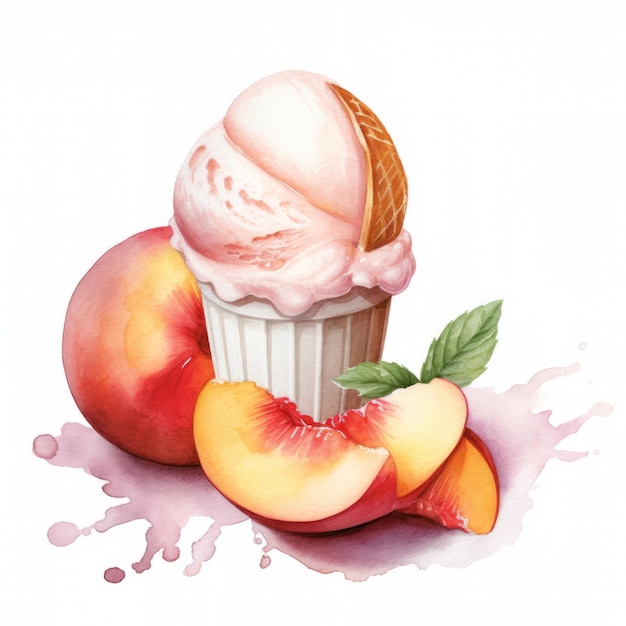This detailed image depicts a painting of a round, white paper cup filled with peach-colored ice cream, emphasizing its unmistakable peach flavor through the peach tones splattered along the base. The ice cream is adorned with a small wafer placed on the side. Surrounding the cup, there is a full peach positioned to the left and three peach slices to the right, with two green leaves nestled between the slices. The bottom of the image is accented with peach juice, reinforcing the peach theme.